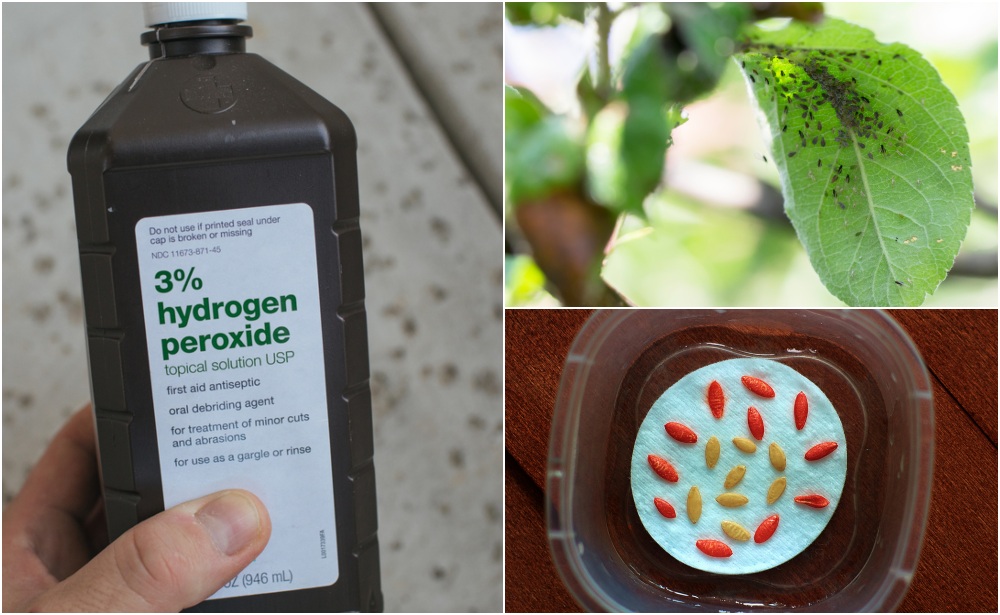The composite image is divided into three sections. The left half features a hand holding a brown bottle with a white cap and a white label that reads "3% hydrogen peroxide" against a grayish background, clearly showcasing the thumb and finger gripping the bottle. The right side of the image is split into two smaller photos. The upper photo displays a green leaf, seemingly outdoors, populated by numerous small black bugs. The lower photo reveals a clear, squarish container with a piece of paper at the bottom, upon which red and yellow seed-like items are neatly arranged. This arrangement appears to illustrate a tip for growing healthy plants, detailing the use of hydrogen peroxide, an infested leaf, and some seed or mineral preparations.